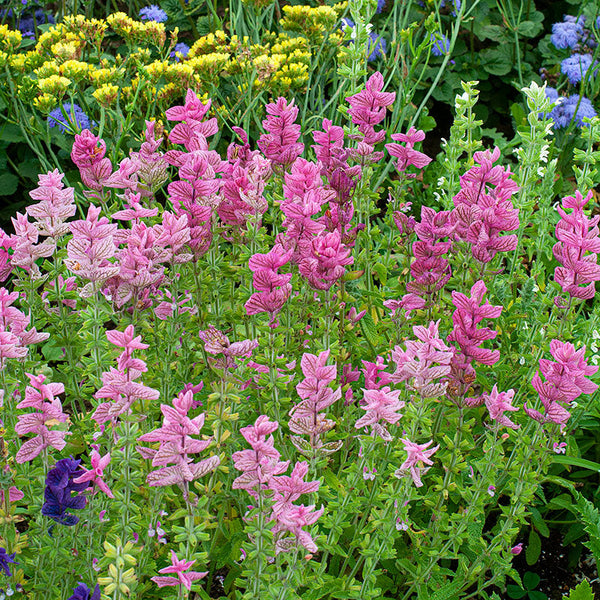This vibrant square-shaped outdoor photo captures a meticulously tended garden bathed in daylight. Central to the image are tall plants with long green stems adorned with green leaves. Atop each stalk blooms a cluster of five or six flowers, showcasing a gradient of pinks from light to dark. Accompanying these are similar plants displaying purple blooms, though fewer in number. Interspersed among these are delicate yellow flowers resembling baby's breath, adding a touch of soft luminosity. Additionally, small clusters of bluish-purple flowers encircle the scene, contributing to the rich tapestry of colors that include verdant greens, shades of pink, yellow, and violet. This harmonious garden tableau, devoid of any text or words, emphasizes the beauty of nature in a cozy, cultivated space.